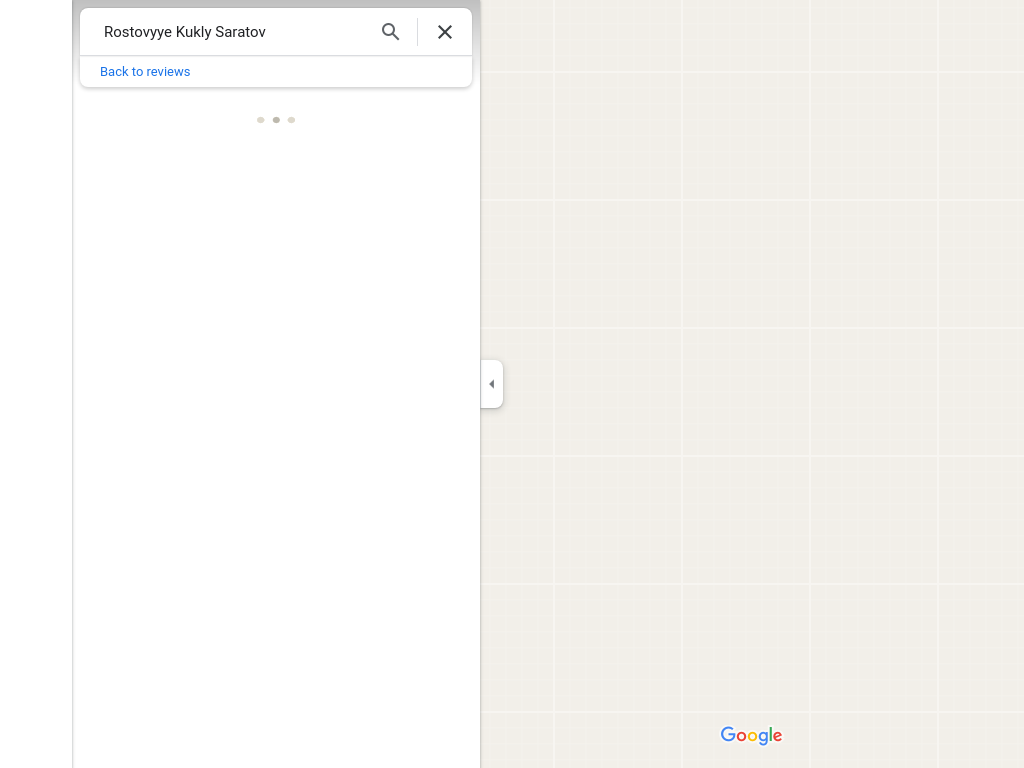A screenshot of a partially-loaded Google Maps interface on what appears to be an Apple device, such as a laptop or desktop. The user is attempting to search for "Rostovyye Kukly Saratov," presumably a location or establishment. Due to low internet speed, the map on the right side of the screen has failed to load, displaying a light, tannish-gray background with a white grid pattern. On the left side, the search bar sits above a white box where search results would typically appear, but it remains empty. Below the search bar, a blue link labeled "Back to reviews" suggests this could be a location with user reviews. The familiar Google logo is visible at the bottom of the map section, confirming that this is indeed the Google Maps interface.